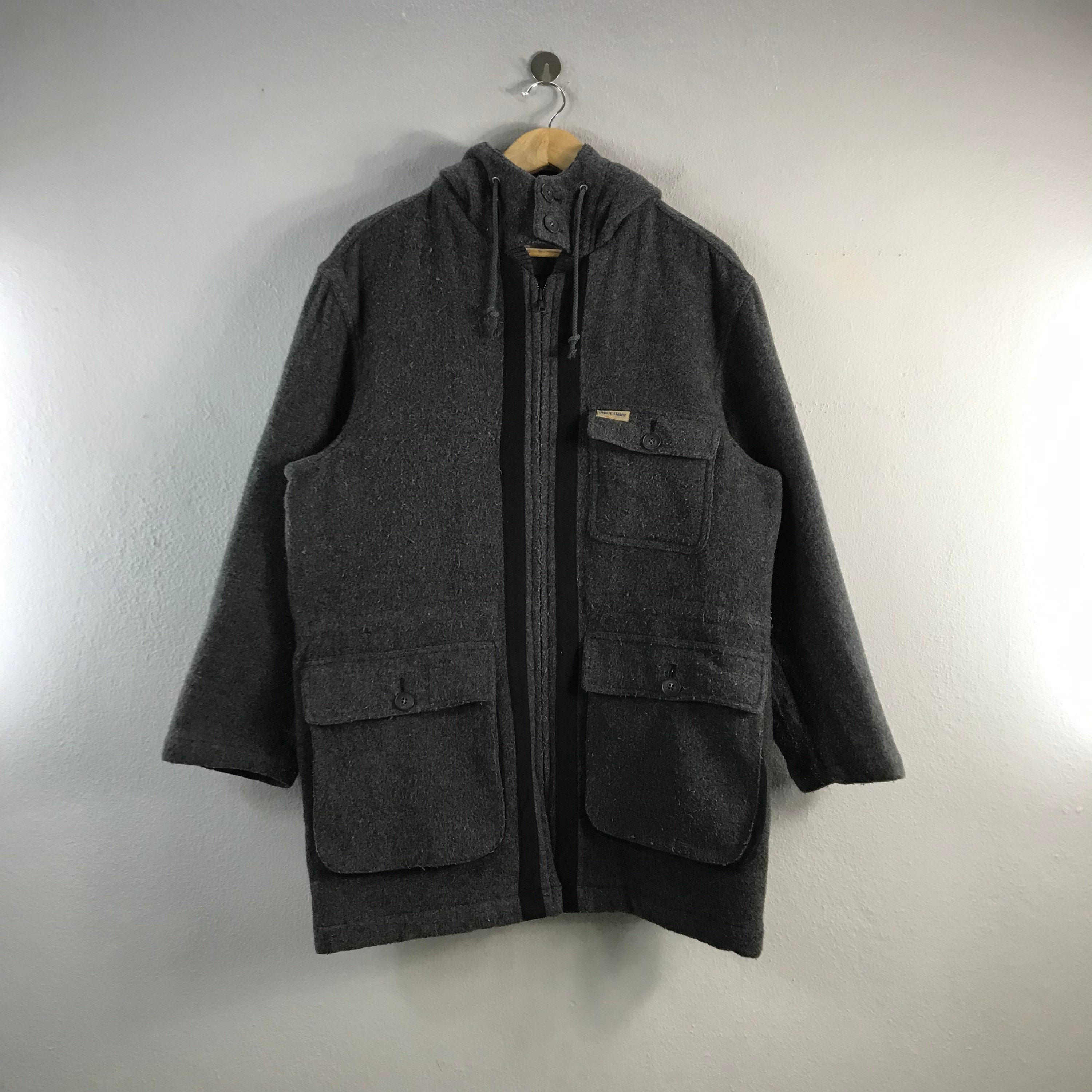This indoor photograph features a gray cotton hoodie jacket with wool-like texture, hanging from a light brown wooden hanger fixed to a gray wall. The jacket, resembling a Carhartt-style workman's jacket, has a zipper running up to its hood, which includes two pull strings. The front showcases three pockets: two large ones at the bottom and a smaller chest pocket on the upper left, labeled with an unreadable yellow tag. Light reflections on either side of the jacket and a flash creating a semi-circular mark on the wall highlight the setting. Long sleeves complete the design, emphasizing its practical and rugged aesthetic.